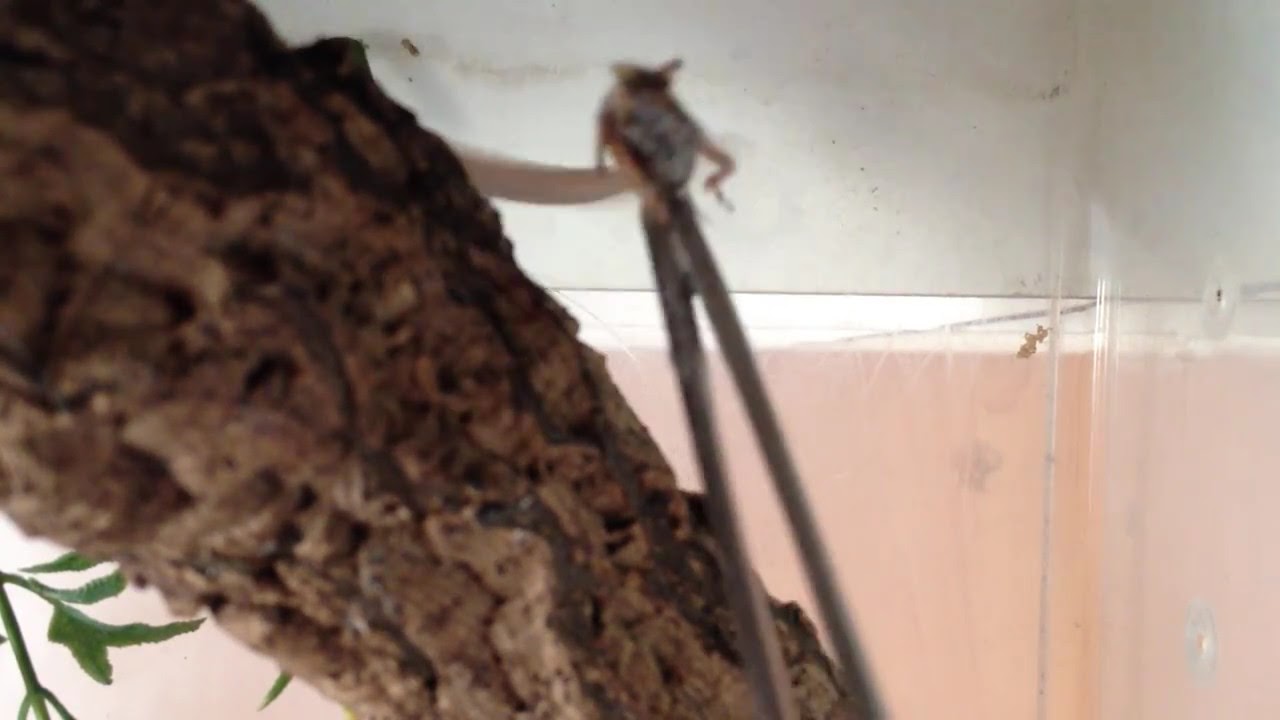In the blurry image taken indoors, we see what appears to be part of a glass aquarium or terrarium. The main focus is a piece of bark or a woody trunk extending diagonally from the top left to about the bottom middle of the image. The wood is thick with deep bark, creating a natural yet indistinct appearance. Attached to the wood is a string extending to the top middle of the image, from which two strings hang downwards towards the center. The left bottom side features a couple of artificial-looking leaves with visible stems. Close to the center, angled towards the right, are two sticks converging to a point, resembling chopsticks. Atop these sticks is a very blurry and uncertain figure, possibly a creature with brownish, curved legs, which could be an insect, rodent, or bird. The background features a light pink and white hue, consistent with the look of plexiglass, adding to the aquarium-like setting.